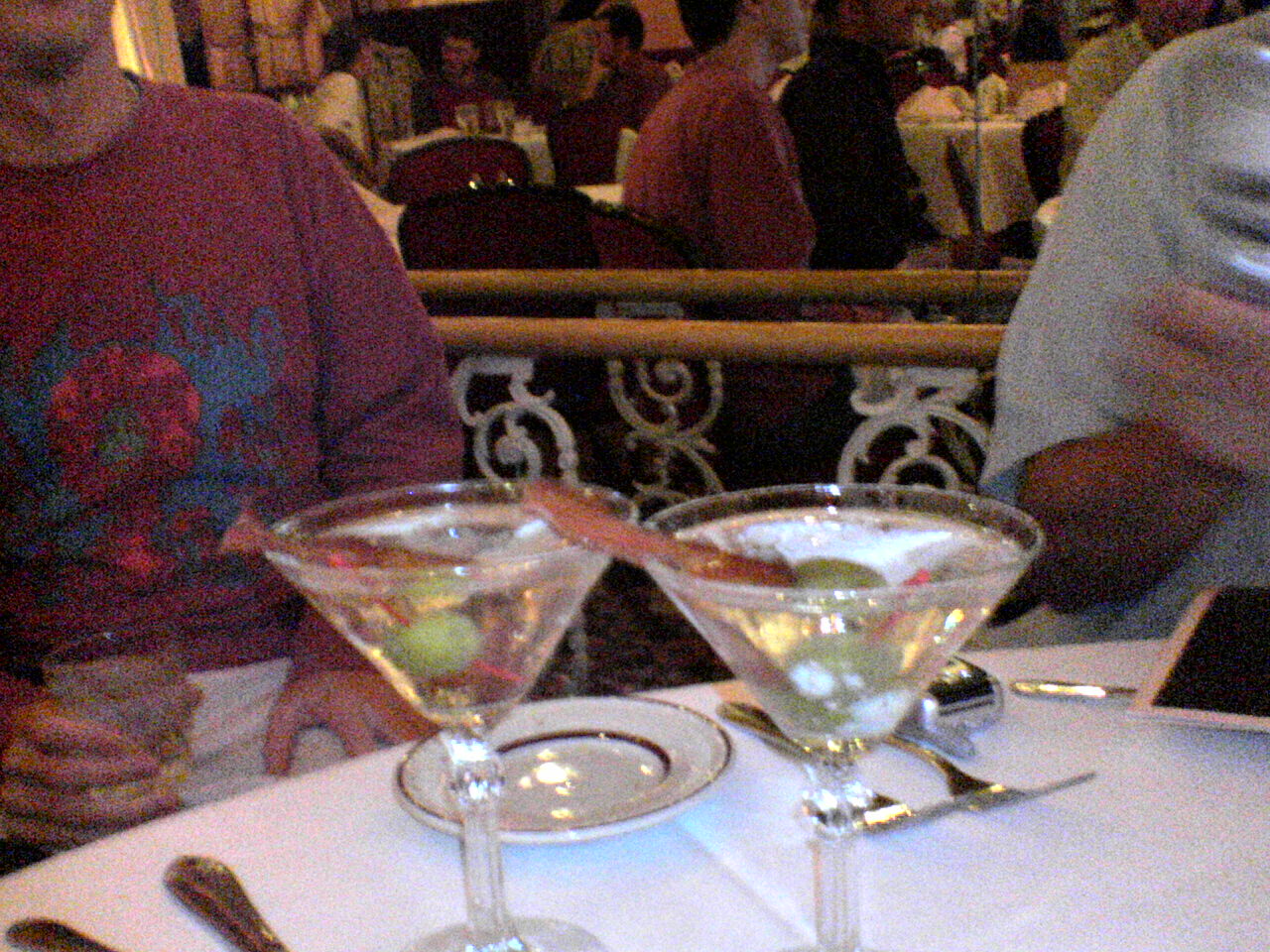This image captures a lively dining scene with two men at a restaurant. The foreground is dominated by a neatly set table featuring a white linen tablecloth, white China plates with gold trim, and an array of silverware including two forks, a spoon, and a knife. In the center of the table, there are two clear martini glasses, each adorned with an olive and what looks like a piece of bacon. To the right, a man in a white short-sleeved shirt appears either clapping or moving his hand, with a square object in front of him that might be an iPad or a menu, and a cell phone. On the left, another man is dressed in a red sweater with blue and red details on the front and white pants; he holds a drink in a whiskey glass. Behind them, a white railing made of decorative iron supports frames the scene, with other restaurant patrons visible in the background, adding to the bustling atmosphere.